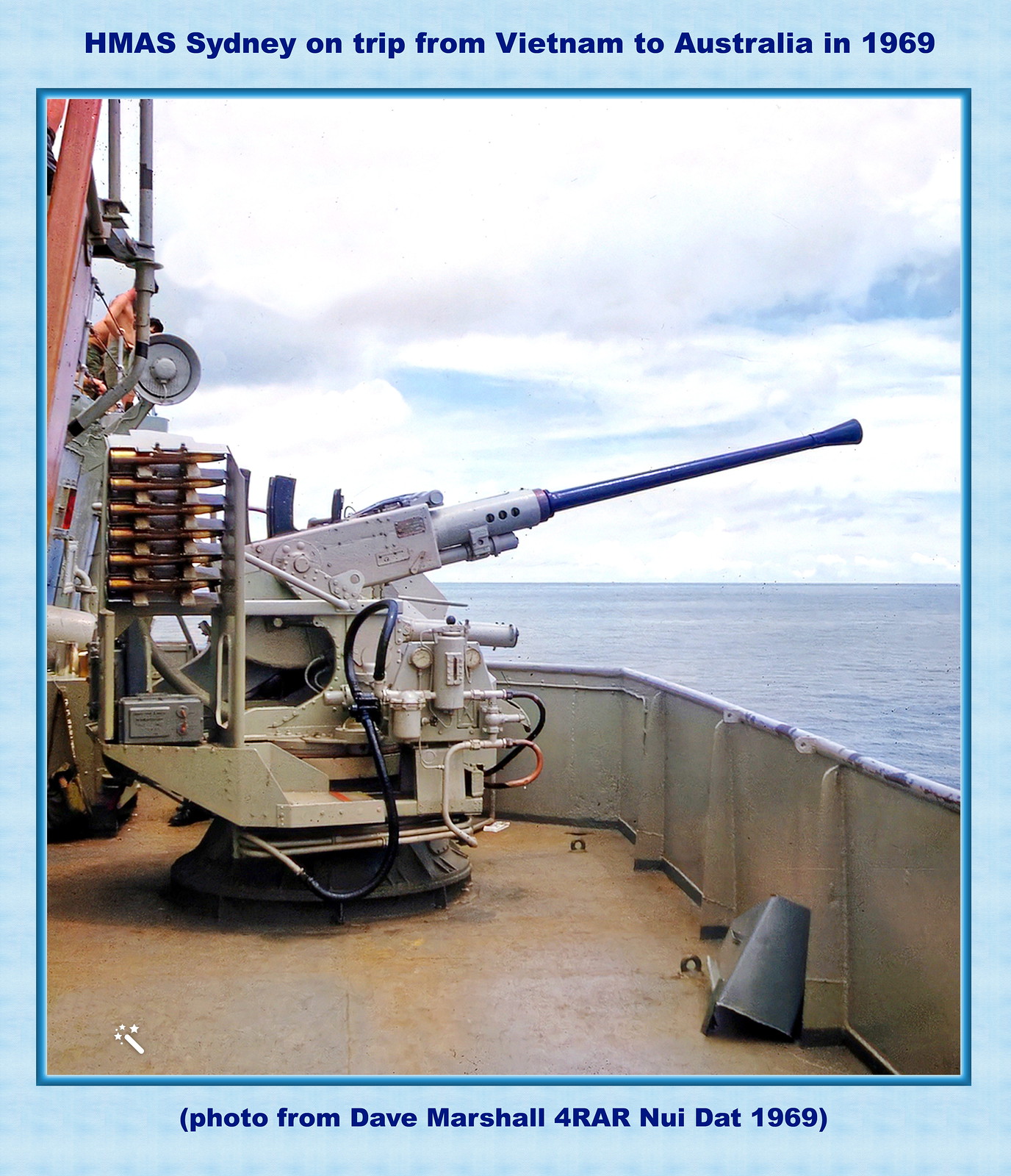The image depicts the HMAS Sydney on its voyage from Vietnam to Australia in 1969, captured in a photograph by Dave Marshall for RAR Nui Dat, 1969. The photo is bordered by light blue with an additional darker blue frame inside, featuring descriptive text at the top and bottom. The scene shows the back right-hand corner of the ship stretching out into the deep blue sea under a hazy, white, and slightly blue sky scattered with grayish clouds. Dominating the lower half of the image is a large, rotatable anti-aircraft artillery gun, poised and focused towards the open sea with a supply of shells visible at its rear. A horn or speaker is noticeable on the left-hand side of the deck. The ship's flat expanse is devoid of any visible crew, giving a serene yet commanding view of the ongoing voyage.